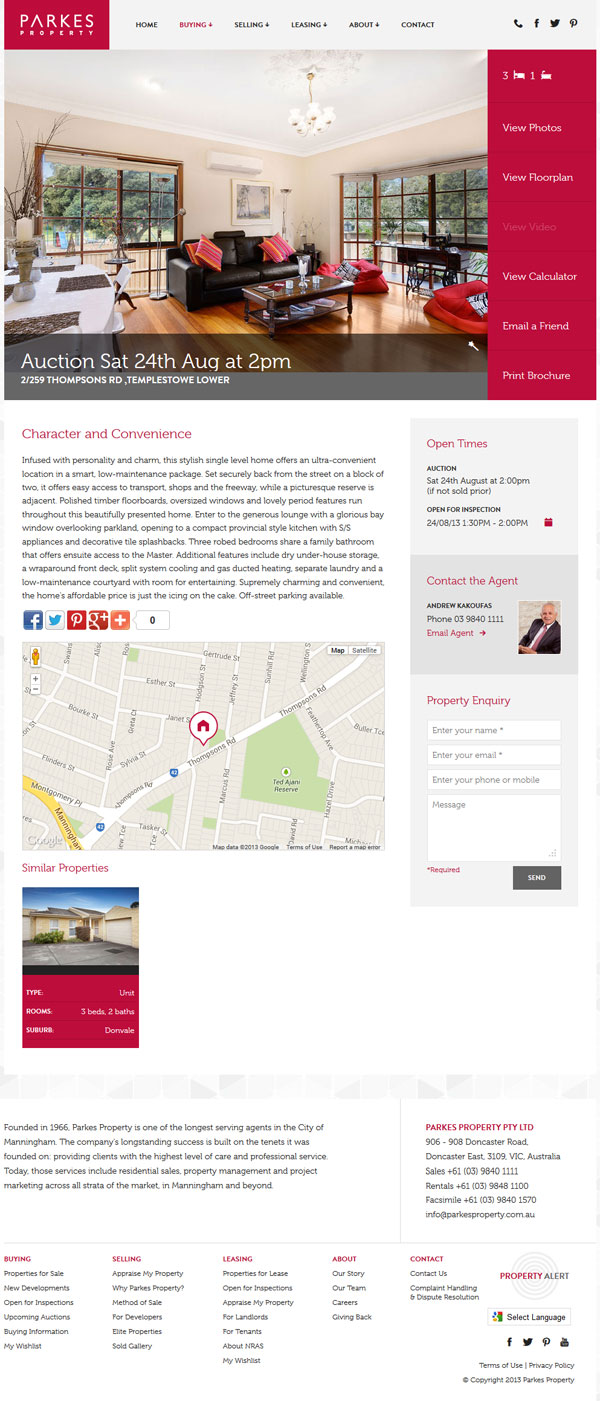This captivating image showcases an elegant property currently listed on the Parks Property website. The photograph features an interior view of a beautifully decorated home with a pristine white backdrop. The room is filled with natural light streaming through large open windows, giving a clear view of the outdoor daytime scenery, which includes an abundance of trees and a neighboring beige-colored house.

Inside, the room is painted in warm beige tones with subtle tulip lights adorning the ceiling. The walls are decorated with tasteful artwork, and the room boasts a hardwood ground floor. The main seating area includes a sleek black leather couch adorned with vibrant striped pillows. A stylish brown wooden coffee table, centered with a vase holding a candle and several decorative items, complements the setting. Another seating option in the room is a plush red bean bag chair, accented with decorative cushions.

An elegant white table with brown placemats is set further into the room, featuring an exquisite centerpiece comprising a candle surrounded by flowers and twigs. This detail enhances the overall sophistication of the space.

The property is set to be auctioned on Saturday, August 24th at 2 p.m. at 21259 Thompson Road, Templestone Lower. An open inspection is scheduled for the same day from 1:30 p.m. to 2 p.m. Prospective buyers can contact the agent, Andrew Koffas, an experienced agent, at 0398401111 or via email through a provided link.

For those interested in learning more about the property, the website offers the ability to enter personal details and message the agent directly. The listing also comes with a map for convenient location tracking and links to connect on various social media platforms including Facebook, Twitter, Pinterest, and Google+, as well as another unspecified orange plus symbol.

Similar property listings are available, reflecting the diversity offered by Parks Property, a well-established real estate agency founded in 1966. This agency is one of the longest-serving in the city of Manningham. Their office is located at 906 to 908 Doncaster Road, Australia, with separate contact numbers for sales, rentals, and facility inquiries, along with a dedicated email address for additional information.